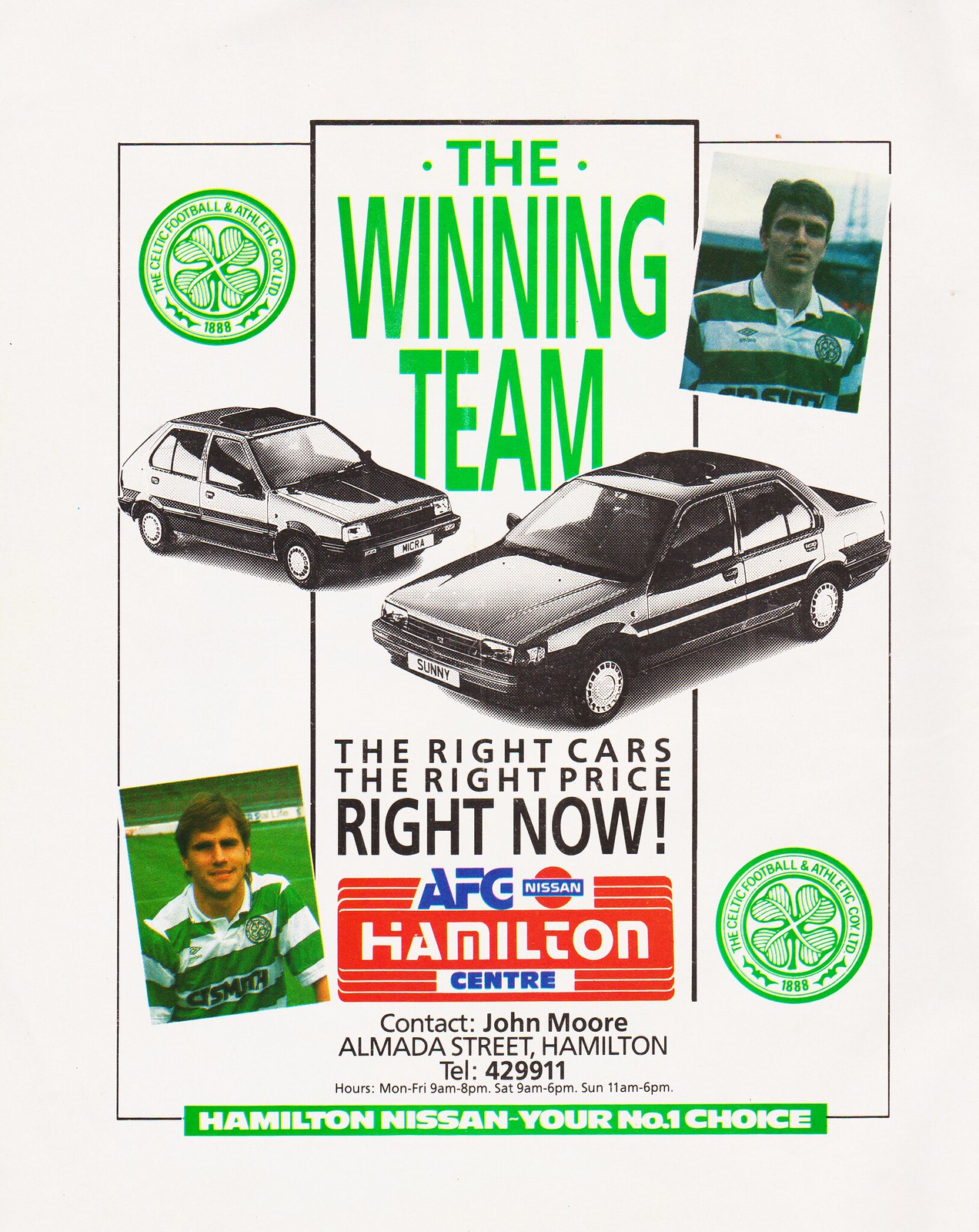The image appears to be a scanned advertisement from an old magazine, featuring a blend of automotive and sports elements. On a tan background, the top left corner prominently displays "The Celtic Football and Athletic Co. Ltd. 1888," accompanied by a four-leaf clover logo. Centrally, large green letters proclaim "The Winning Team," flanked by detailed black-and-white sketches of two 1980s-style sedans. To the right of the caption is a photograph of a soccer player wearing a green and white horizontally striped jersey, mirrored by another such image in the bottom left. Beneath the car sketches, the advertisement reads, "The right cars, the right price, right now. AFG Nissan, Hamilton Center," followed by contact details for John Moore at Almada Street, Hamilton. It signs off with "Hamilton Nissan, your number one choice." Additional color details include shades of black, green, white, gray, red, and blue, suggesting this page was part of a sports magazine’s advertisement section.